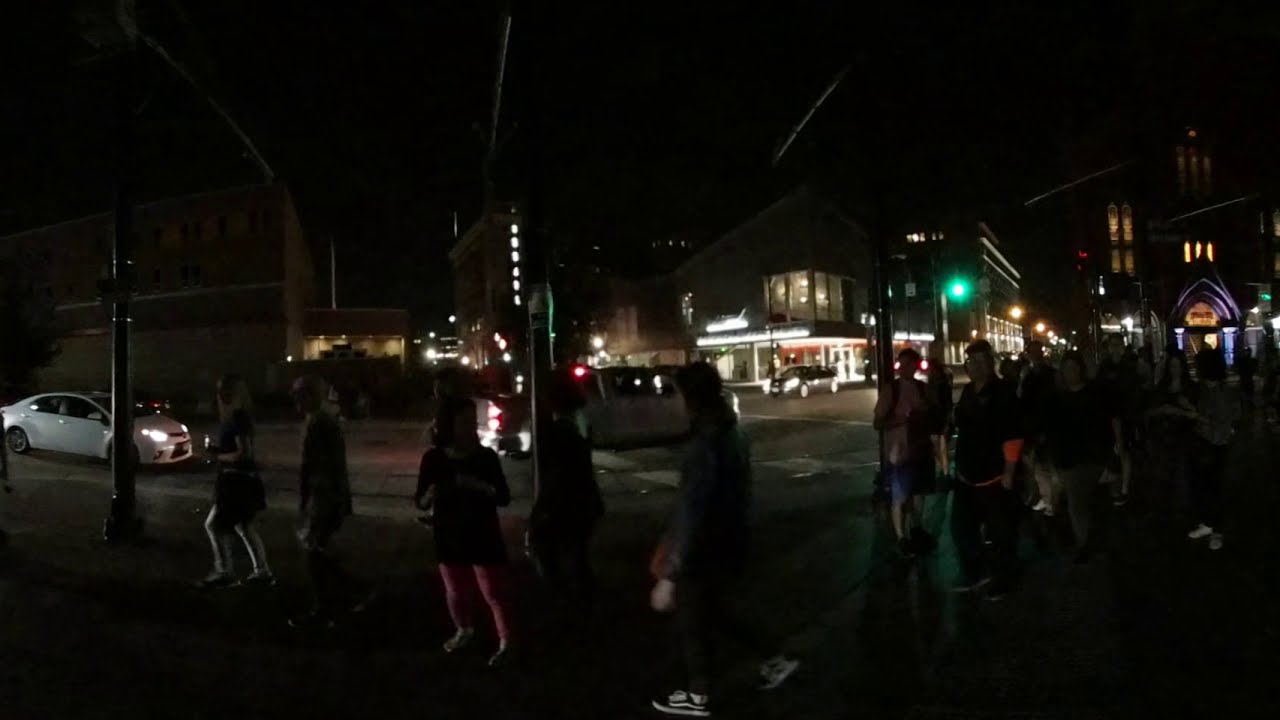The nighttime photo captures a dark city street scene illuminated by scattered lights from buildings and vehicles. The central focus is on a crowd of people, some moving towards and others walking away from the camera, casually dressed with a person in sneakers visibly prominent in the center. To the left, a white sedan with its headlights on drives along the road, which features visible green and red traffic lights. The right side and background showcase a larger, more dispersed crowd near an arched door with stained glass windows, possibly a church entrance. Behind this scene, well-lit buildings, including what looks like a restaurant, cast various lights and shadows, adding to the bustling yet dimly lit atmosphere.